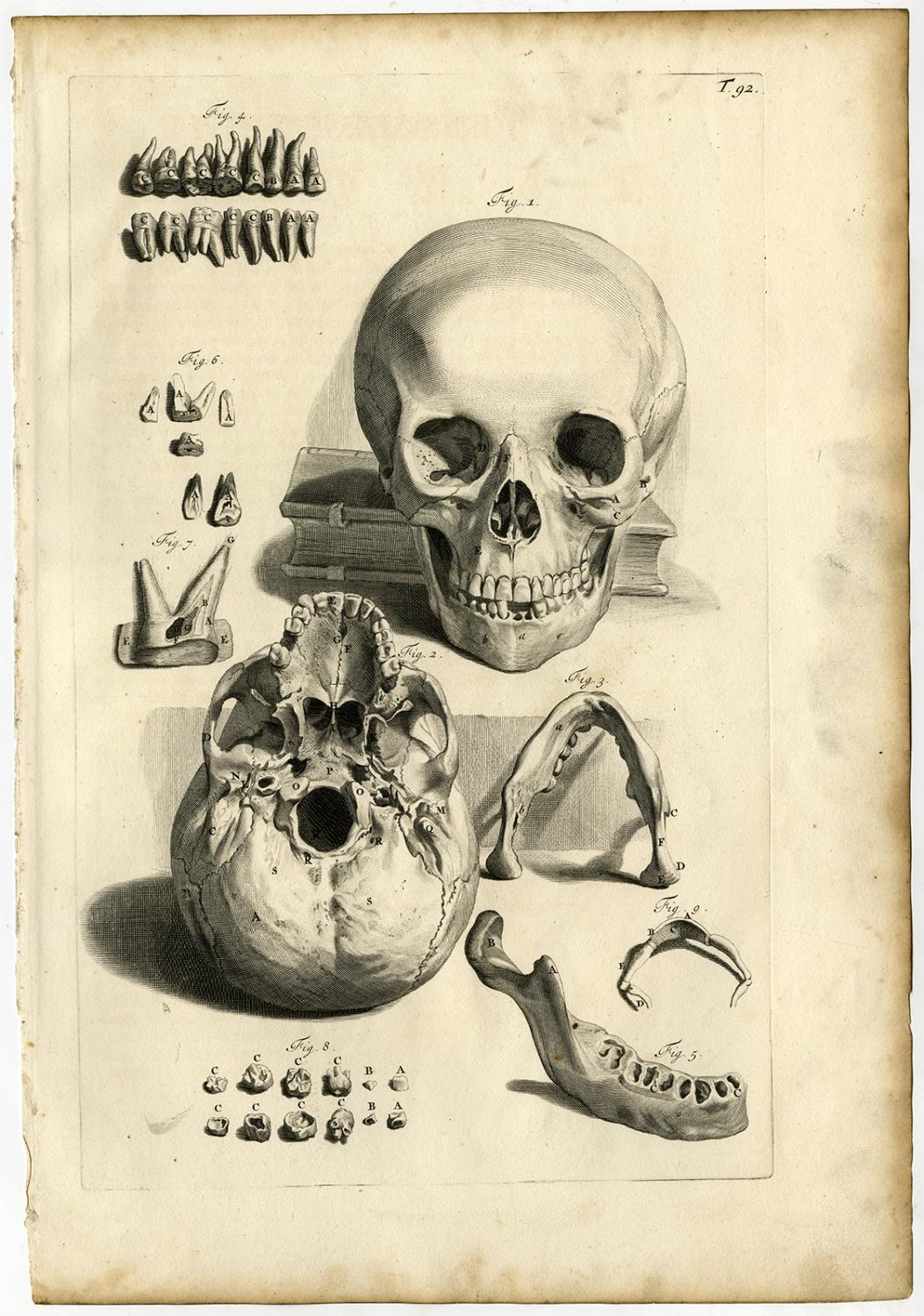This detailed black and white illustration, rendered on weathered and yellowed paper with smudged and dirty edges, depicts multiple views and components of a human skull and its teeth, identified and labeled for educational purposes. At the center of the image, the primary skull faces directly towards the viewer, resting atop an old book with its spine turned away, obscuring the title. Beneath this skull, another view displays the skull from the bottom, highlighting the openings, including where the spinal cord enters. This reversed view exposes the internal structures such as the sinus cavities. The jawbone is detached and parts of it, along with an array of teeth labeled A, B, C, and D, are scattered throughout the illustration. In the top left corner, two rows of teeth are arranged, showing both the front and root views, while additional close-ups and cross-section diagrams of teeth populate the bottom left and right sections. Each segment of the drawing, including the various skull and jaw perspectives, and the individual teeth, is denoted by figure numbers. The top right of the drawing bears the text "TG2," further identifying the illustration. This comprehensive drawing provides a meticulous and somewhat unsettling depiction of human skull anatomy and dental variation.